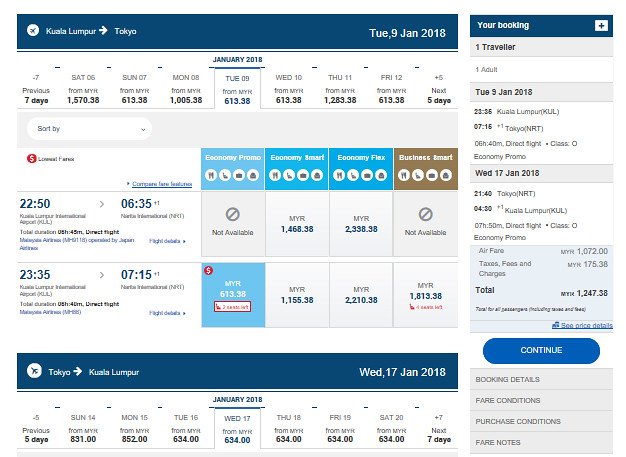The image presents a dark blue banner at the top divided into two sections. On the left side, the banner displays "Kuala Lumpur" (capitalized as K-U-A-L-A L-U-M-P-U-R) with an arrow pointing to the right, leading to the word "Tokyo" (capital T-O-K-Y-O). On the right side, the banner indicates "2 TUE 9 JAN 2018," designating Tuesday, 9th January 2018.

In the center of the image, "January 2018" is prominently displayed. Below it, several entries are listed, providing financial data and dates:
- "-7 Previous 7 Days: Set 06 from M-Y, $1,570.38"
- "7 Days from M-Y: $613.38"
- "Monday, 08 from M-Y: $1,005.38"
- "Tuesday from M-Y: $613.38"
- "Wednesday: $613.38"
- "Tuesday from M-Y: $1,283.38"
- "Friday from M-Y-K: $613.38"

The information continues with a note: "+5 for the next 5 days."

Below this section, there's a table labeled "Lowest Fares," showing different fare options:
- Economy Promote
- Economy Smart
- Economy Flex
- Business Smart